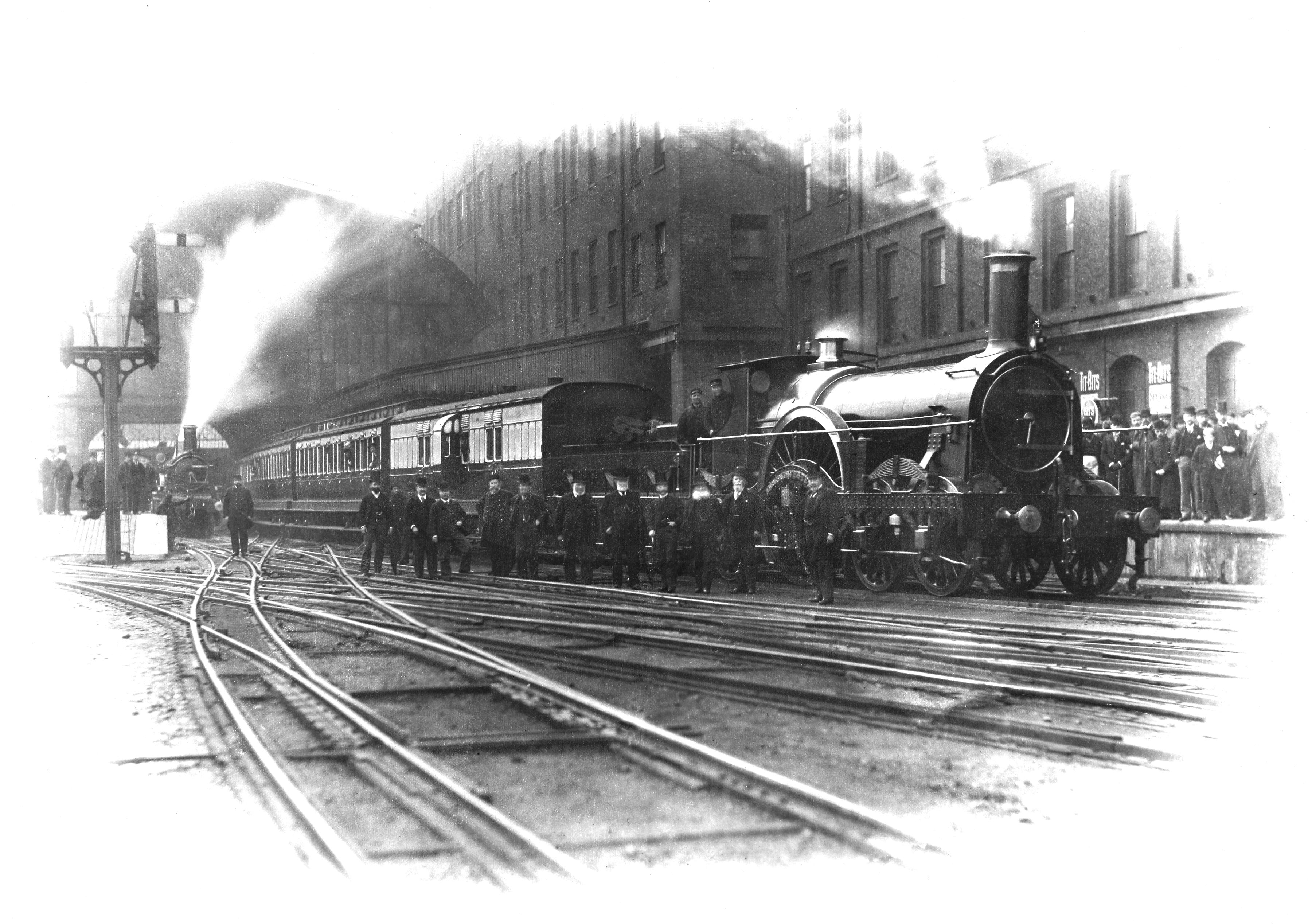In this 1920s era black and white photograph, a group of about ten men is posing next to a steam-emitting train, dressed in classic attire of the period—black suits, hats, and a few with long bushy beards. The men stand on train tracks with a series of buildings and a tall structure with many windows possibly serving as the train station in the background. The scene suggests a bustling atmosphere, as another train is visible to the left, also releasing smoke, with more men dressed similarly standing nearby. The image captures the essence of a traditional time when train travel was commonplace, accentuated by the presence of tracks stretching across the scene and additional onlookers standing on the raised walkway beyond the trains.